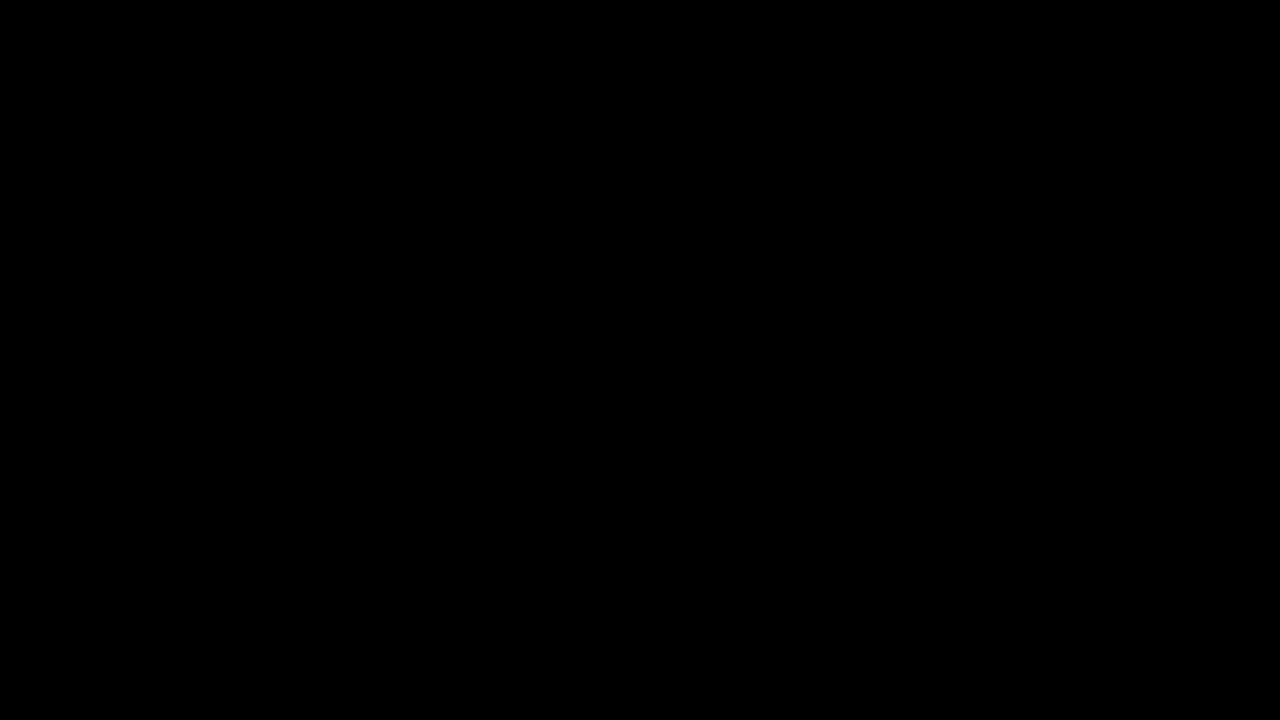The image is a completely dark, solid black rectangle in a landscape orientation. There are no objects, text, or people visible. The entire screen is uniformly black with no discernible shapes or forms, making it impossible to determine any specific setting or scene. The photo is characterized by its absolute darkness, void of any lighter shades or variations, and appears as though it could serve as a backdrop due to its blank, featureless nature. The only visible detail is the uninterrupted expanse of black that fills the entire frame.